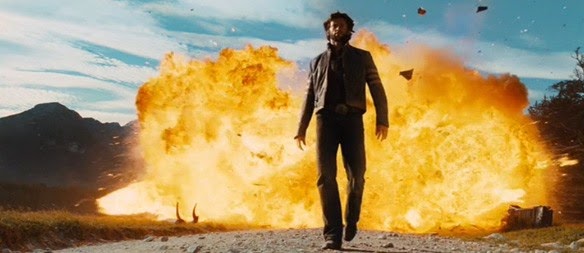This is a detailed still shot from the movie "Wolverine Origins," capturing Hugh Jackman walking away from a massive explosion. Jackman is in the forefront, dressed in a long-sleeved, dark leather jacket—either brown or black—and black jeans. His black curly hair and beard frame his face, although detailed facial features are hard to make out. His arms are spread out, exuding a sense of maximum coolness as he strides away from the blast without looking back. 

The explosion behind him is immense, dominating most of the background with its vibrant hues of orange, yellow, and white. Scattered debris, some appearing as small brown pieces, is visible in the air. To the right of the explosion, the silhouette of a few trees comes into view, while on the left, a mountain range can be faintly seen in the far distance.

Jackman is walking on a gravel road, speckled with patches of grass and composed of grayish-brown dirt, sand, and rocks. The sky above is blue with scattered fluffy white clouds, adding a serene contrast to the fiery chaos below. Hills and trees pepper the distant landscape, completing the dramatic scene.